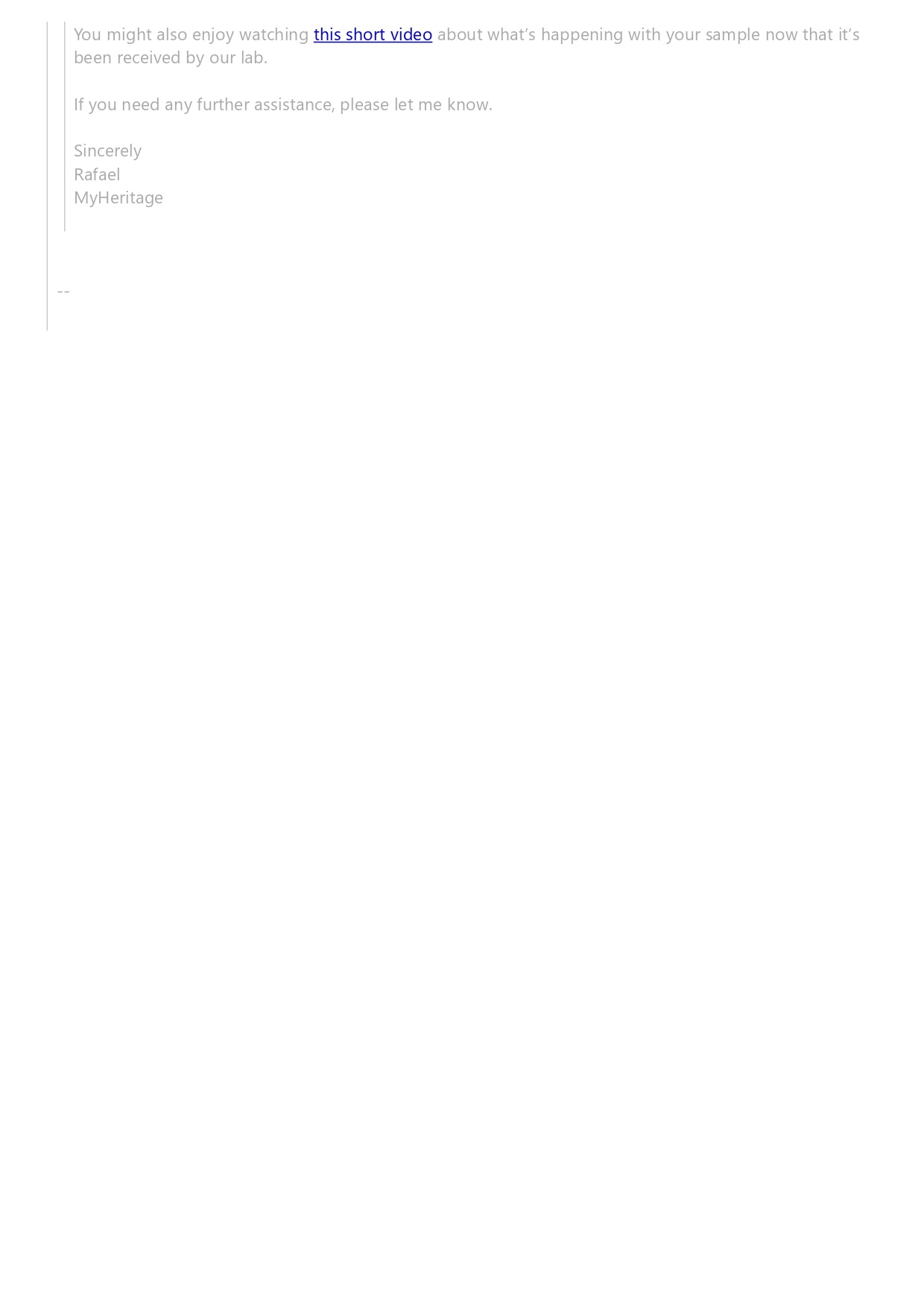**Descriptive Caption:**

The image appears to be a partial screenshot of a website communication, potentially an email or a message from a customer service portal. The background and text are rendered in light gray, giving a soft, muted appearance to the elements on the screen. 

At the top, two thin gray lines frame the main message, with one line starting from the top of the communication and extending slightly past it, followed by a small space and another thin gray line below. These lines visually segment the content, adding a subtle structure to the communication layout.

The primary text reads, "You might enjoy watching this short video about what's happening with your sample now that it's been received by our lab." The phrase "this short video" stands out in blue-colored font and is underlined, indicating it is a clickable hyperlink.

Below this, another sentence provides an option for further assistance: "If you need further assistance, please call." The communication concludes with a polite closing: "Let me know. Sincerely, Raphael." Following this, the signature "My Heritage" appears, all in the same light gray font, and the text is aligned to the left.

The content is divided into three distinct sections:

1. Information about the video link.
2. Offer of further assistance.
3. A cordial farewell and signature.